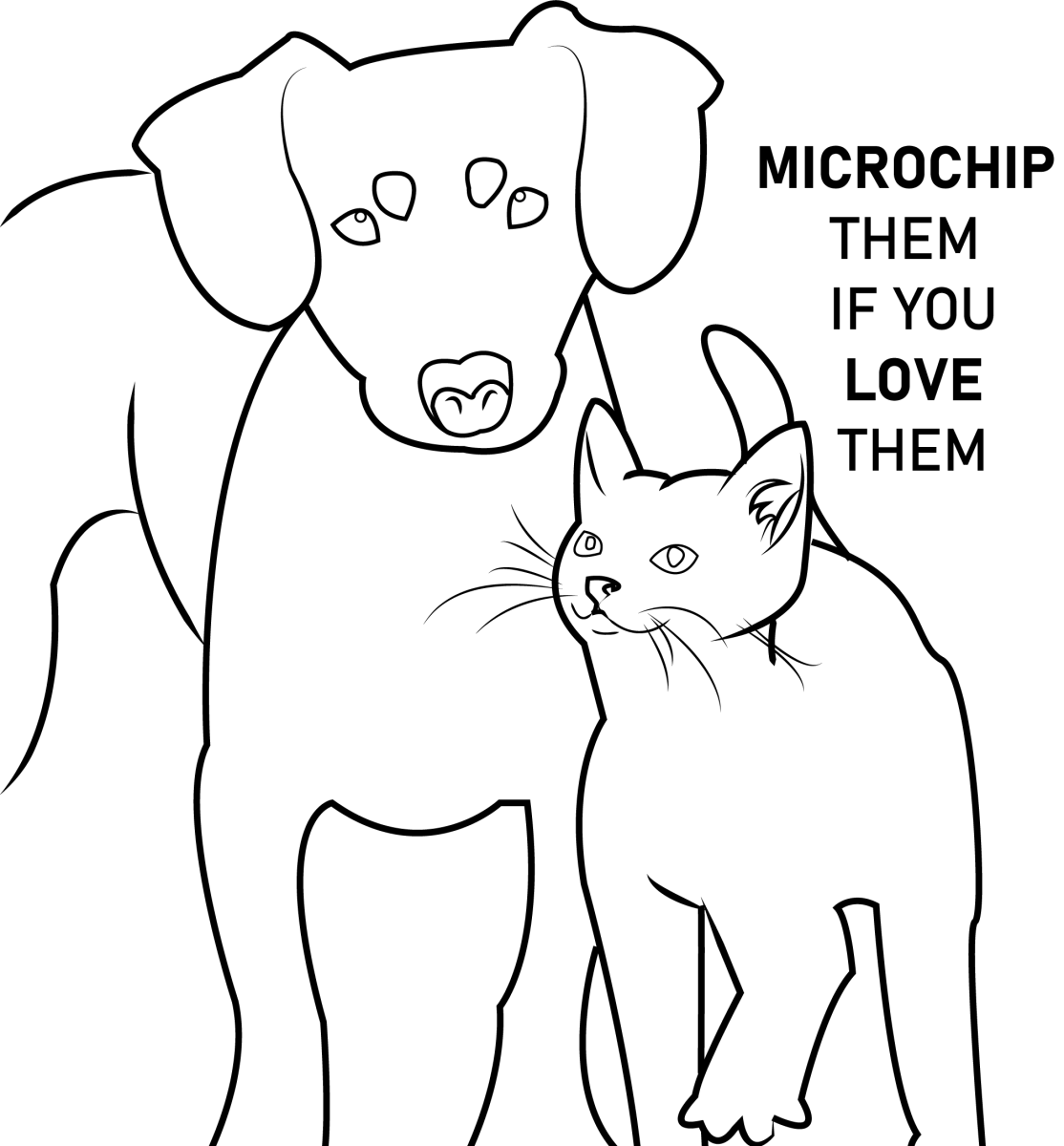The black and white drawing is a rough, yet well-executed, pencil sketch intended as an advertisement mock-up. It features a short-haired dog and a domestic cat, both outlined with some filled-in details like the whiskers and eyes. The small dog is facing forward, gazing slightly cross-eyed upward, presumably at its owner. Beside the dog, the cat is rubbing against it while looking up with a slight smile and lifting its right paw. Both animals are devoid of collars and presented in a frontal view. Above the animals, in the upper right-hand side of the image, the text reads, "Microchip them if you love them," with the words stacked on separate lines: "Microchip" at the top, followed by "them," "if you," "love," and "them" at the bottom. The overall effect is a charming, though simple, hand-drawn illustration designed to emphasize the importance of pet microchipping.